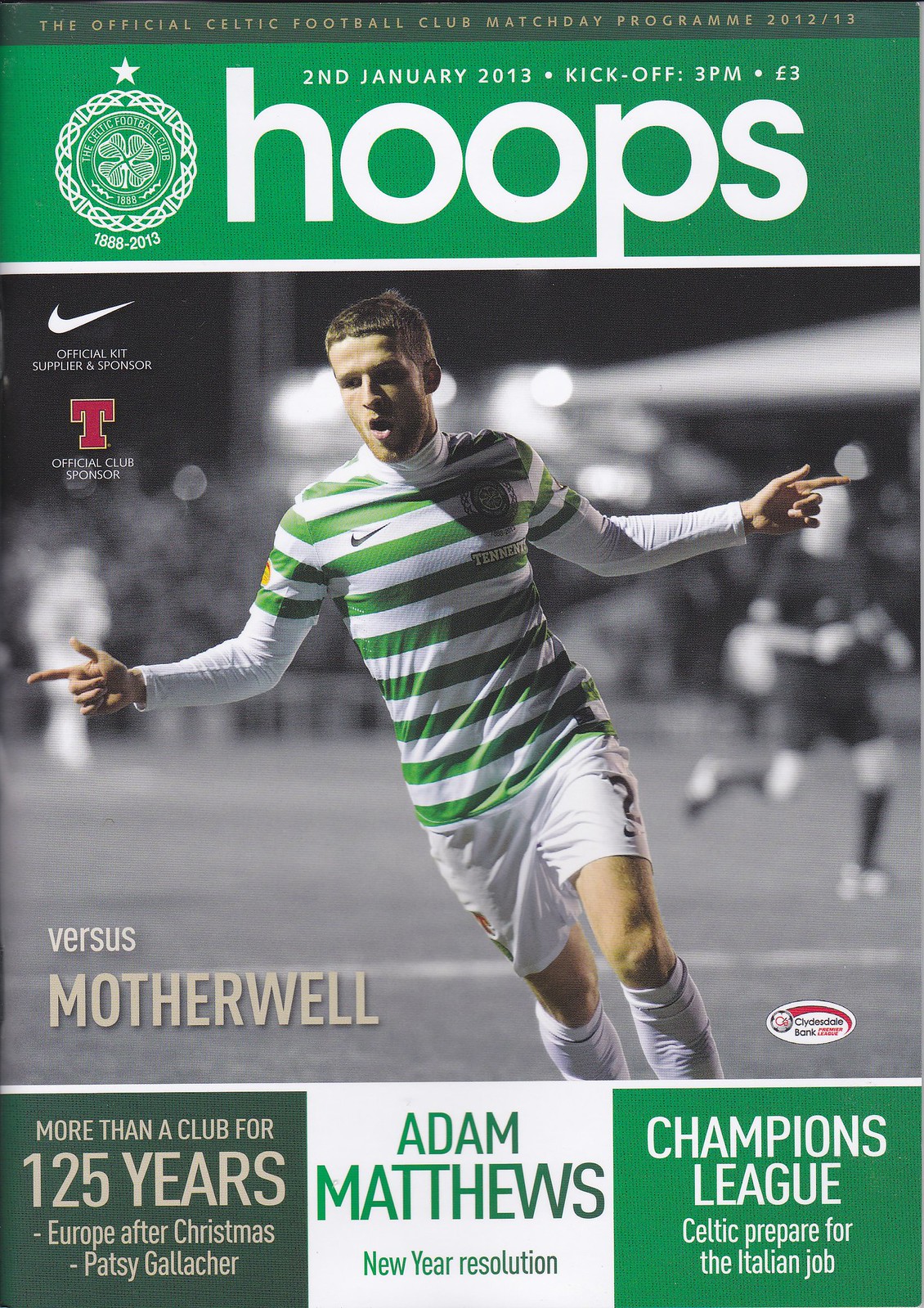The rectangular advertisement image is an official Celtic Football Club matchday program for the 2012-2013 season. It prominently features a photograph of a soccer player in mid-game action, wearing a green and white striped Nike jersey, white shorts, shin guards, and tall socks. Above the player, the text reads "The Official Celtic Football Club Match Day Program 2012-2013," and includes the match details: "2nd January 2013, Kickoff 3 p.m., $3 or €3." To the right of this text is the word "Hoops" accompanied by the Celtic FC logo, which features a four-leaf clover encircled by Celtic knots, the numbers "1888-2013," and a star on top.

Below the central photograph, a Nike check mark signifies their role as the official supplier and sponsor, just above a large red "T" indicating the official club sponsor. The bottom of the picture bears the text "Versus Motherwell." The lower section contains three informational blocks: the first highlights the club's longevity with "More than a club for 125 years," followed by "Europe after Christmas" and "Patsy Gallacher." The second block mentions "Adam Matthews' New Year resolution." The third provides a competitive note with "Champions League: Celtic prepare for the Italian job."